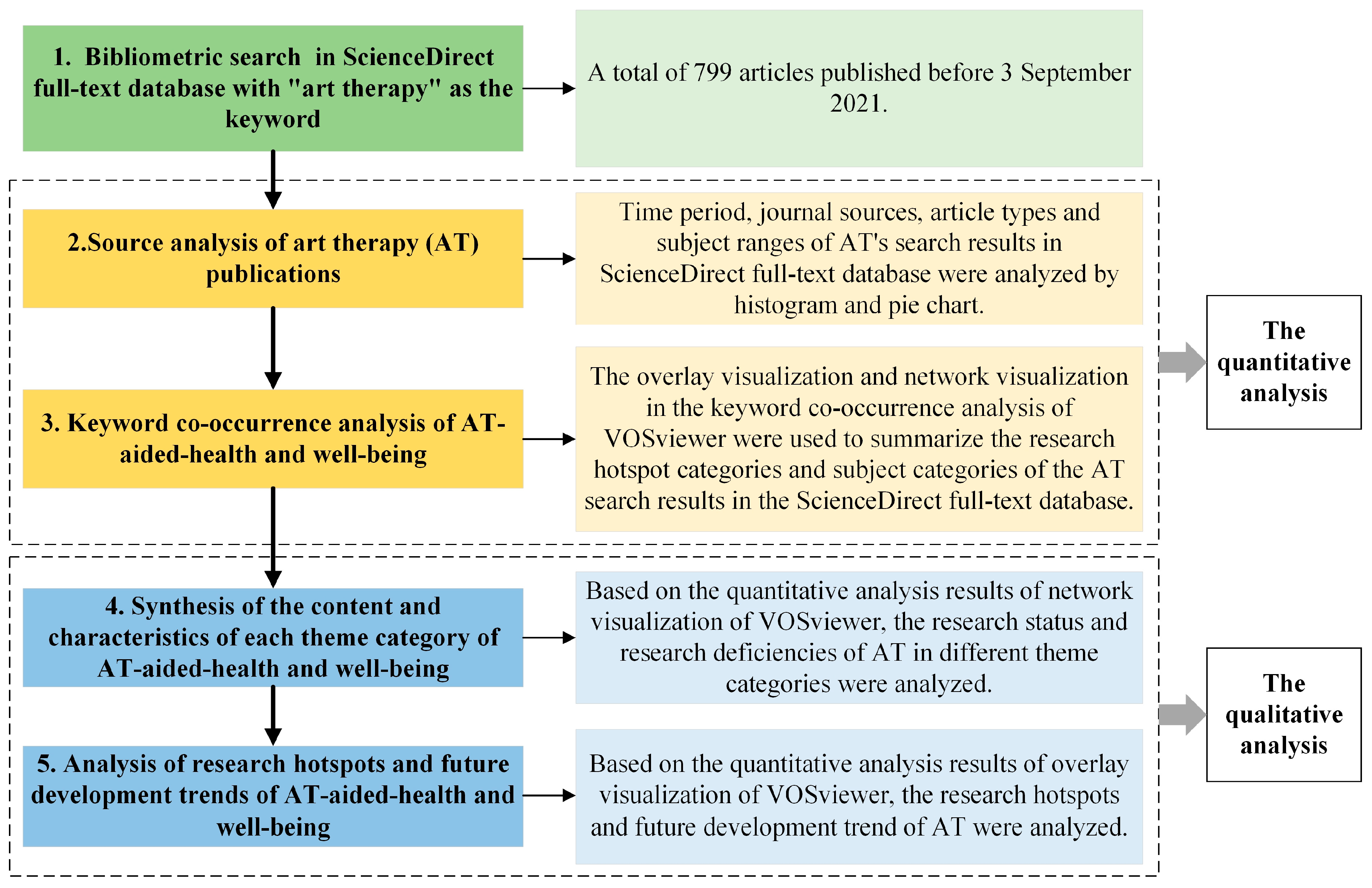This diagram depicts a detailed bibliometric analysis workflow for "Art Therapy" as a keyword within the Science Direct Full Text Database. The left column consists of five colored rectangles: starting with a green box at the top followed by two yellow boxes and two blue boxes. Each of these boxes contains black or dark gray text summarizing various stages of the analysis. 

1. **Green Box**: Bibliometric Search and Science Direct Full Text Database with "Art Therapy" as a Keyword.
2. **Yellow Box**: Source Analysis of Art Therapy (AT) Publications, providing further details on the time period, journal sources, article types, and subject ranges derived from the AT search results.
3. **Yellow Box**: Keyword Co-Occurrence Analysis of AT-Aided Health and Well-Being.
4. **Blue Box**: Synthesis of the Content and Characteristics of Each Theme Category of AT-Aided Health and Well-Being.
5. **Blue Box**: Analysis of Research Hotspots and Future Development Trends of AT-Aided Health and Well-Being.

From each of these boxes, arrows point rightward to lighter-colored, corresponding boxes that provide additional qualitative and quantitative analysis. The arrows also point downward from each box to concurrently follow the sequential analysis steps.

On the right, directly corresponding to each numbered box on the left:
1. **Green Box**: Details of the total number of articles published between September 3, 2000, and September 3, 2021.
2. **Yellow Box**: Histogram and Pie Chart Analysis of Time Period, Journal Sources, Article Types, and Subject Ranges of the AT Search Results.
3. **Yellow Box**: Visualization of Research Hotspots and Subject Categories using VOS viewer in the Keyword Co-Occurrence Analysis.
4. **Blue Box**: Analysis of Research Status and Research Deficiencies of AT based on Network Visualization Results.
5. **Blue Box**: Analysis of Research Hotspots and Future Development Trends of AT based on Overlay Visualization Results.

Additionally, the yellow boxes have a dashed outline indicating quantitative analysis, while the blue boxes likewise signify qualitative analysis. Two extra boxes on the right provide additional summarized insights, maintaining the structure of quantitative (yellow) and qualitative (blue) assessments. The complex interplay of arrows illustrates a structured progression from initial search to detailed analysis, both vertically and horizontally.